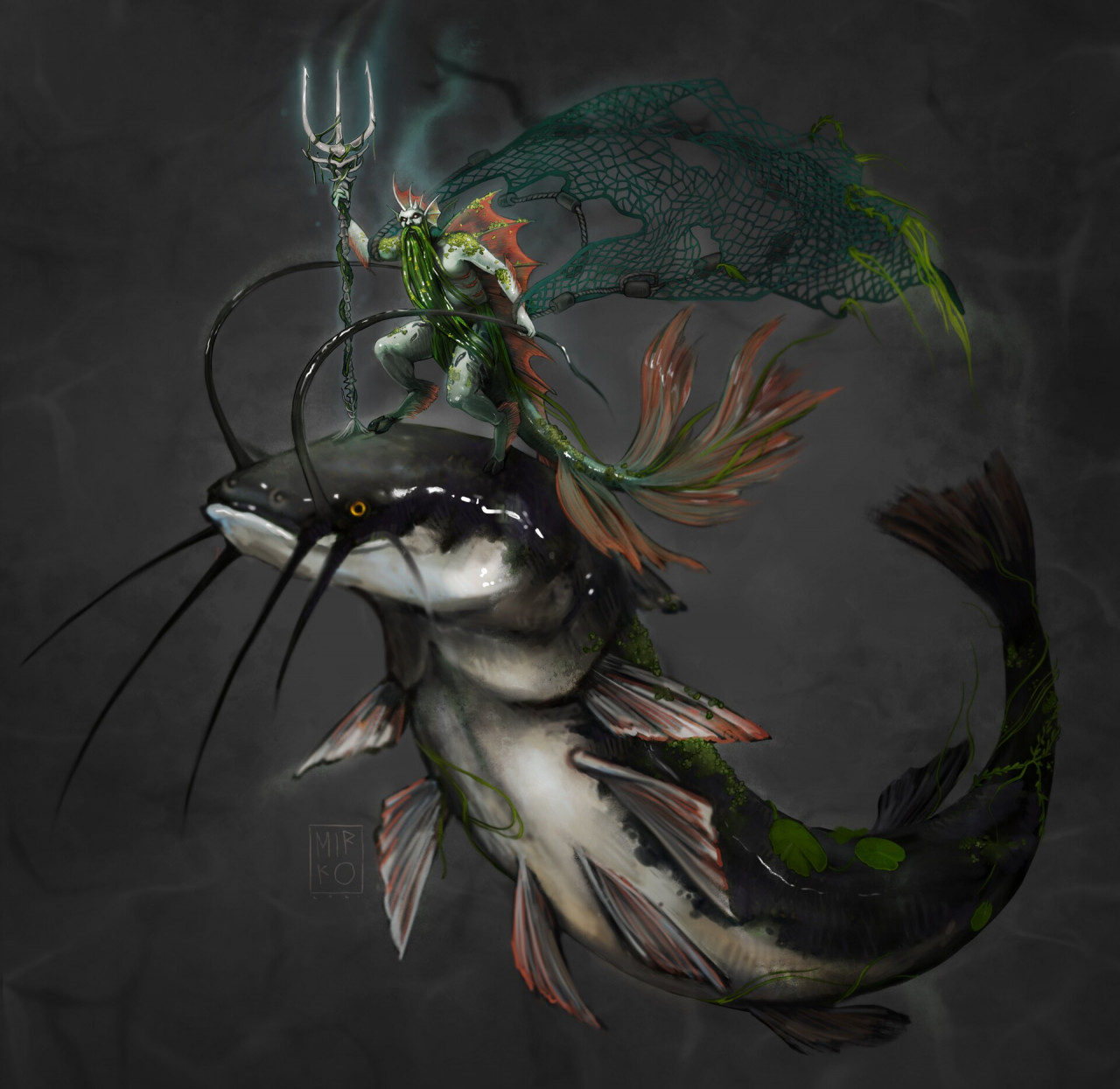The image is a detailed, square, multi-color artistic print set against a gray background with no border. At the center, there is a colossal catfish-like creature. Its body arches upward, with a primarily black top adorned with green spots and a white underbelly. This extraordinary fish has six front fins, numerous antenna-like whiskers, and hints of red along its body. 

Atop this mythical fish stands a humanoid sea-man figure, blending human, goat, and aquatic traits. The figure's defining features include a long, algae-like green beard, bat-like wings, and a fin structure with pinkish hues on his back. He wields a black and green trident with white prongs in one hand and a green net in the other. The humanoid’s lower half features a green tail adorned with pinkish-white appendages. The illustration is rich with fantastical elements, emphasizing the surrealistic fusion of marine and mythological motifs.